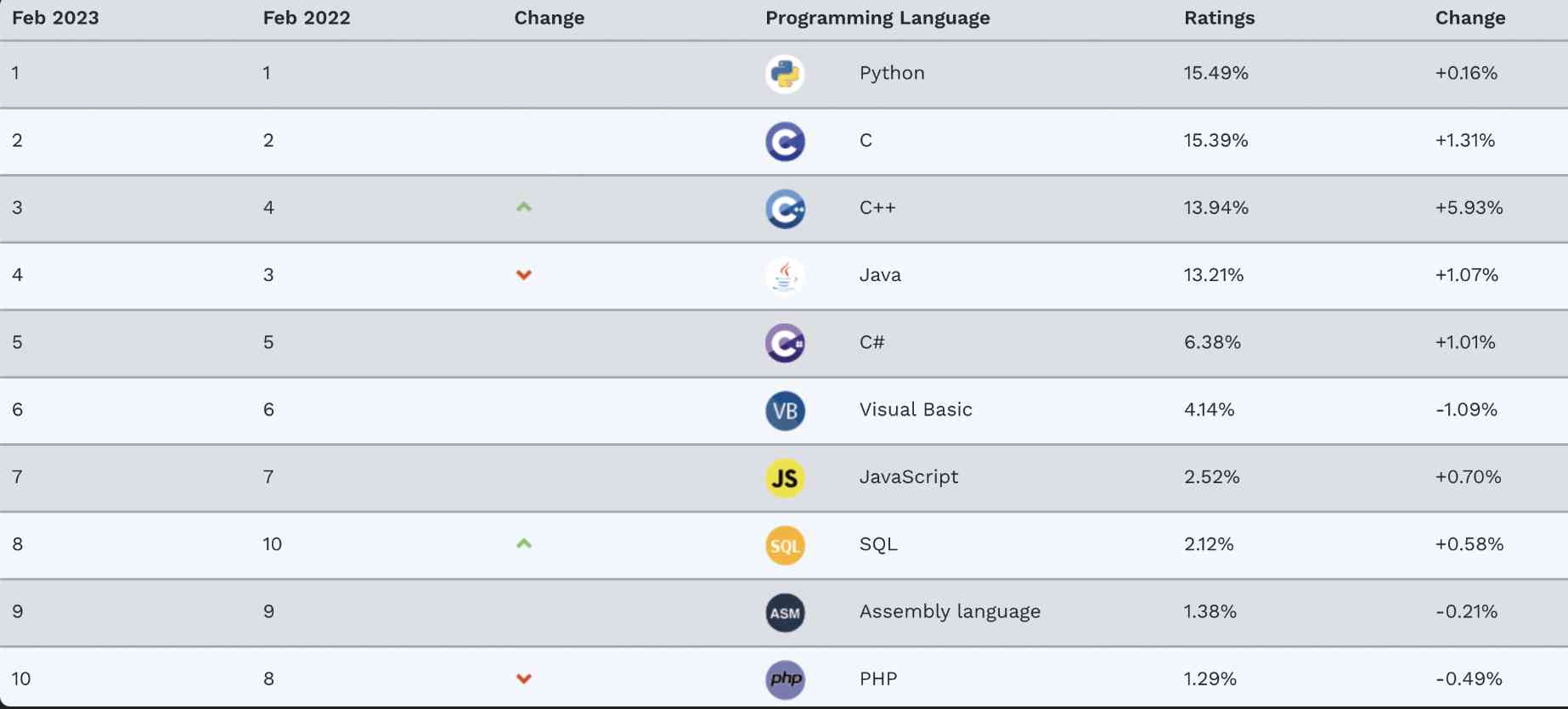**Detailed Caption for Image: Programming Language Popularity Table**

This image depicts a comparative table of programming language popularity ratings for February 2023 and February 2022, along with the changes recorded over the year. The table is organized with the following columns: **Dates**, **Programming Language**, **Ratings (% Feb 2023)**, **Change (%)**.

- **Dates**: The top of the table lists "February 2023" and "February 2022" to indicate the time periods being compared.
- **Programming Languages**: The programming languages ranked from 1 to 10 for February 2023 are: Python, C, C++, Java, C#, Visual Basic, JavaScript, SQL, Assembly Language, PHP.
- **Ratings for February 2023**: The corresponding ratings percentages are:
  1. Python - 15.49%
  2. C - 15.39%
  3. C++ - 13.94%
  4. Java - 13.21%
  5. C# - 6.38%
  6. Visual Basic - 4.40%
  7. JavaScript - 2.52%
  8. SQL - 2.12%
  9. Assembly Language - 1.38%
  10. PHP - 1.29%
- **Change (%)**: The column indicating the change in percentage from February 2022 to February 2023 includes:
  - Python: +0.16%
  - C: +1.31%
  - C++: +5.93%
  - Java: +1.07%
  - C#: +1.01%
  - Visual Basic: -1.09%
  - JavaScript: +0.70%
  - SQL: +0.58%
  - Assembly Language: -0.21%
  - PHP: -0.49%
 
Indicators for changes are shown with green arrows for positive changes and red arrows for negative changes:
- **Green Arrows (Positive Change)**:
  - Programming Languages 3 (C++), 4 (Java), 8 (SQL), and 10 (PHP) show gains in their ratings.
- **Red Arrows (Negative Change)**:
  - Programming Languages 6 (Visual Basic), and 9 (Assembly Language) display losses in their ratings.

Overall, this table provides a clear and detailed comparison of the rating changes for the top 10 programming languages from February 2022 to February 2023, reflecting trends in programming language popularity over the past year.